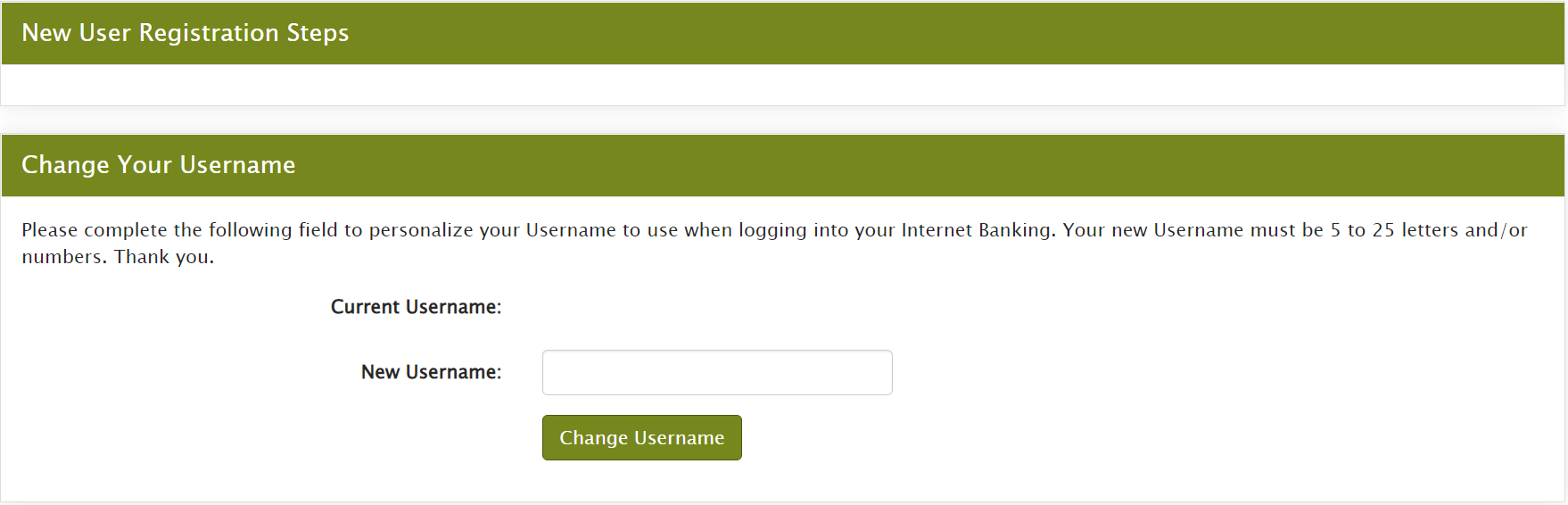This screenshot from my website features a prominently olive green banner at the top in varying shades of bright and deep olive. The banner displays the title "New User Registration Steps" in white text, with each significant word's initial letter capitalized (N, U, R, S).

Beneath this is a white space followed by another identical olive green banner. This second banner reads "Change Your Username," similarly capitalized (C, Y, U). Underneath, in black text, the instructions read: "Please complete the following field to personalize your username for logging into your internet banking. Your new username must be 5 to 25 letters and/or numbers." The word "numbers" is expressed as numerals.

Further down, the form fields are labeled "Current Username" and "New Username." There is an input box beside the "New Username" field. Below this input box, within another green banner, is the button labeled "Change Username" in white text.